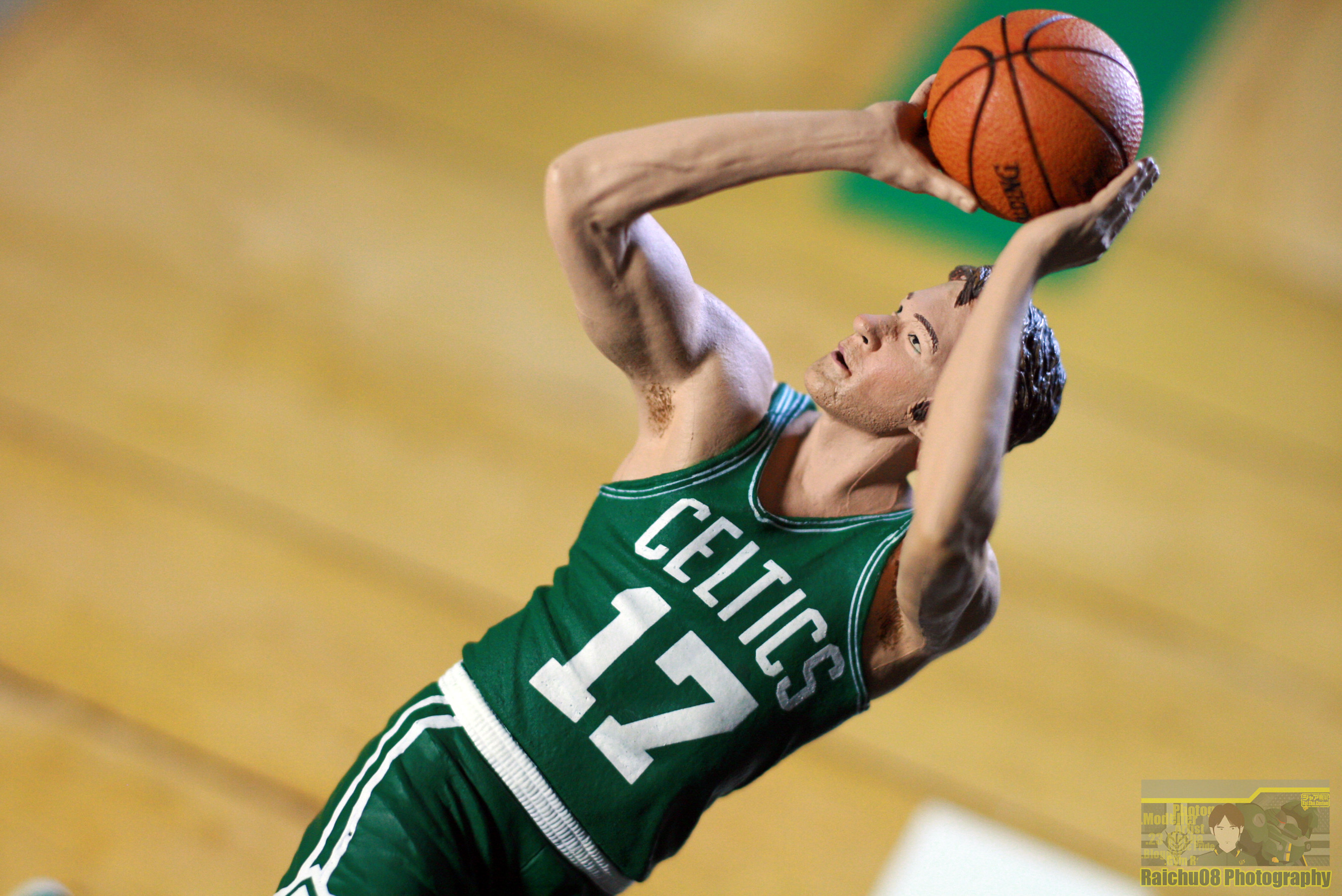The image depicts a figure of a basketball player in mid-action, preparing to make a shot. The player is dressed in a green and white Celtics jersey emblazoned with the number 17 and the word "Celtics." He has light brown hair and holds a brown basketball with both hands. The figure appears to be airborne, poised to throw the ball. The background is blurry, mixing shades of beige, light brown, and green, leaving the setting indistinct but suggesting the floor of a gymnasium with its light wood color. The bottom right corner of the photograph is marked with the text "Rachel 08 photography."